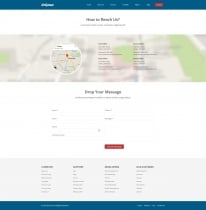Screenshot of a Low-Resolution Webpage: The screenshot, though unclear, shows a webpage with various elements. At the top, a dark blue navigation bar houses several links and a call-to-action button on the right. Below the navigation bar, there is a header section featuring a map. Directly underneath the header, there appears to be a contact form, identifiable by input fields and a prominent red button. The main content of the page is displayed in black text on a white background. At the bottom, a footer section is visible with a light gray background and a dark blue footer bar beneath it.